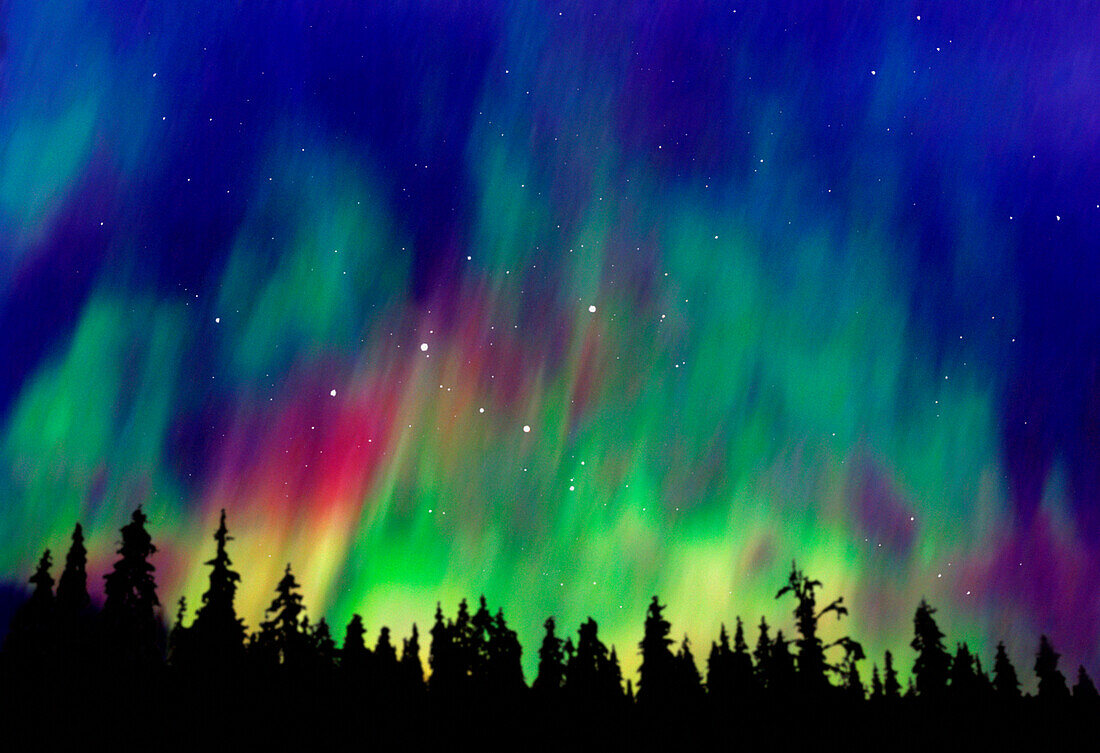This photograph showcases a mesmerizing view of the Northern Lights, with three-quarters of the frame dominated by the enchanting display. The night sky serves as a deep blue backdrop, dotted with twinkling stars. Amidst this celestial canvas, the aurora’s vivid colors – neon green, red, orange, yellow, and touches of blue – create flowing, motion-blurred patterns that intensify at the center near the bottom and gradually fade toward the edges. The lower portion of the image features a silhouette of tall evergreen trees, likely pines, adding a stark contrast to the luminous dance above. The interplay of colors, with neon green being the most prominent, brings vibrant light to the scene, making the photograph a stunning capture of this rare natural spectacle.